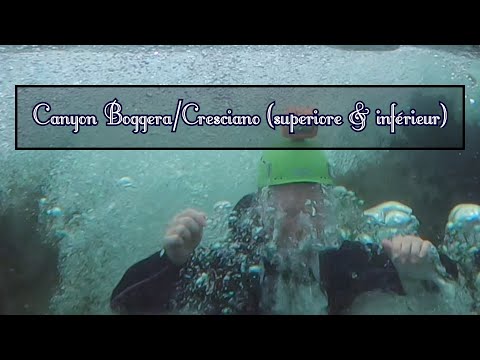The image features a submerged man wearing a black outfit and a green helmet, possibly engaging in an underwater activity. He is surrounded by numerous white and green bubbles, which obscure most of his face, and has a GoPro camera, with a pink mount, on his head. His hands are clenched in fists, seemingly pushing towards the surface. The photograph is framed with black borders on the top and bottom and contains text in a white transparent box with a black border, reading "Canyon Bagheera, Cristiano, Superiore, and Inferior." There are indistinct shapes that might be silver rock formations to the right, adding to the underwater scene's complexity.